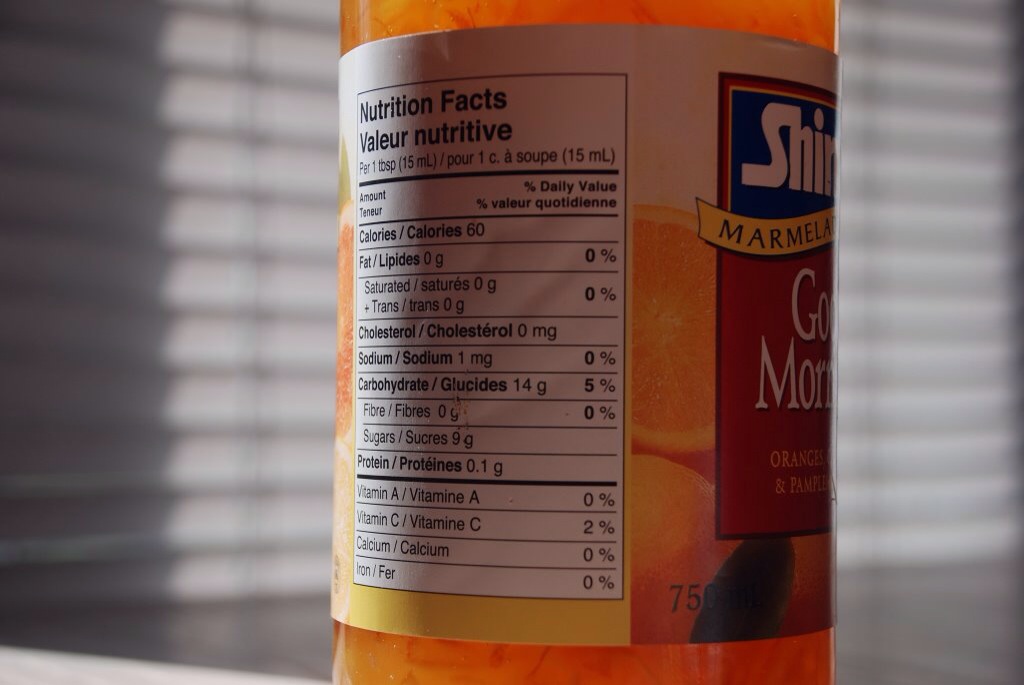The image depicts a glass bottle of marmalade prominently placed on a table. The label of the marmalade bottle reads "Good Morning" and features illustrations of oranges, indicating the citrus fruit flavor. The bottle itself appears orange, likely due to the marmalade inside rather than the color of the glass. The nutritional information on the label specifies that each tablespoon of the marmalade contains 60 calories. The background of the image shows a window with closed blinds, allowing minimal light to filter through from the left side, casting a subdued light over the scene.